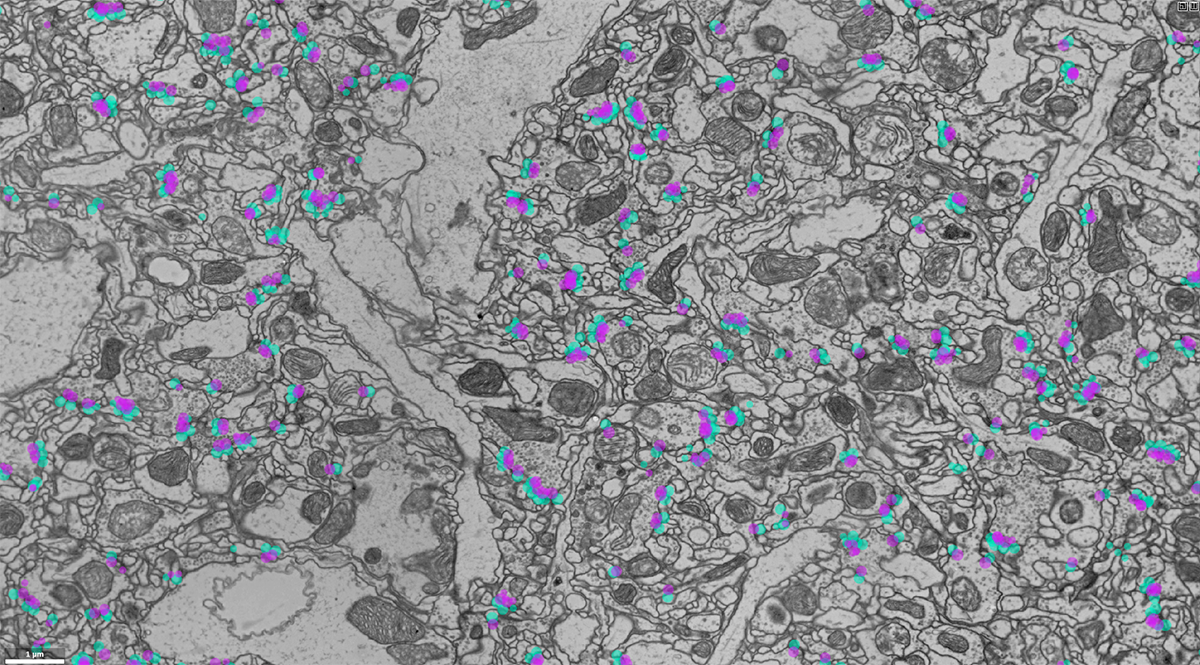This image is a colored drawing, resembling a topographical map, captured within a horizontal, approximately 6-inch wide by 3-inch high rectangular frame without a border. The predominant background features varying shades of light gray, with patches appearing near the top, to the left of center, and descending slightly past the midsection, alongside additional spots of light gray towards the bottom left. The rest of the image is characterized by darker grays, alongside outlined shapes, with highlights of blue and purple colors dispersed throughout.

The composition can be divided into three quadrants, starting with the upper left quadrant, which contains a dense area of drawings, punctuated in the middle by a thin strip descending vertically. The lower left quadrant mirrors this complexity, and adjacent to it, slightly to the right, another slim light gray strip appears. The right side of the image is predominantly a mix of darker grays, shapes, and sporadically placed light blue and purple hues.

The image features hand-drawn elements like oblong shapes and circles, some filled with dark gray. Repeated patterns of bright purple-pink centers, encircled by vibrant greenish-blue tones, are scattered throughout, suggesting an up-close view of a cellular system, though its exact nature is unidentified. A small, thin white horizontal rectangle appears in the lower left corner, with "1PM" inscribed just above it, adding a final touch to this intricate and colorful representation.